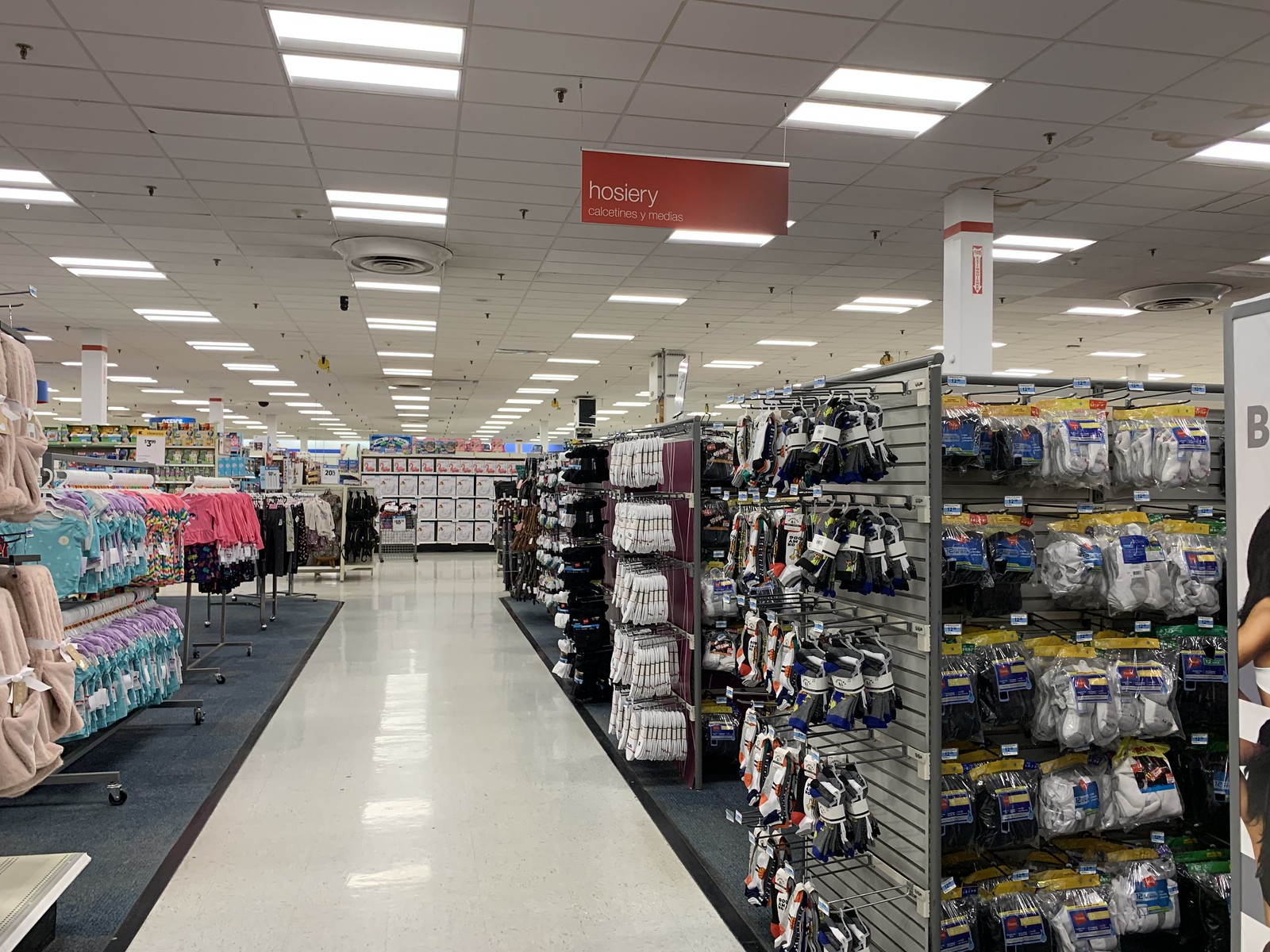This photograph depicts the interior of a large department store, closely resembling the layout of a Walmart. The spacious aisle is lined with glossy white tiles, reflecting the overhead lighting from the white-tiled ceiling with fluorescent lights in parallel lines narrowing in perspective towards the back wall. On the left side of the broad aisle, there's a department dedicated to children's clothing. It features a variety of outfits including racks of blue garments, and in front of them, longer light pink ensembles, possibly bathrobes or dresses. Further in the background, there are racks displaying black pants paired with pink sweatshirts, and against the distant wall, a series of storage bins. To the right of the aisle, prominently marked by a red 'Hosiery' sign with white lettering, are numerous rows of socks and underwear. The department on either side of the aisle is carpeted in a combination of blue and gray, adding a cozy contrast to the bright, reflective aisle.